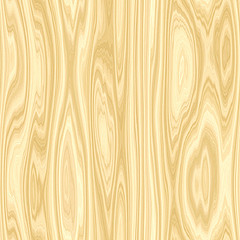The image is a small, square artist's rendition of a piece of synthetic wood, either 3D generated or created through an art program. The wood texture features vibrant and exposed grain patterns, with heavy knotting evident throughout. The coloration varies from light white and light tan to darker shades of tan and a light brown, creating a blend of vertical stripes and circular swirls that emanate from the knots. The grain appears almost too perfect, suggesting the synthetic nature of the image rather than natural wood grain. On closer inspection, the right side of the wood may reveal a face-like pattern formed by the knots, with two eyes and an open round mouth, while the rest of the texture showcases a wave-like pattern and expanded areas where the wood grain seems to unfold from its center. The overall effect is an intricate and detailed imitation of wood, giving an impression of natural beauty despite its manufactured origins.